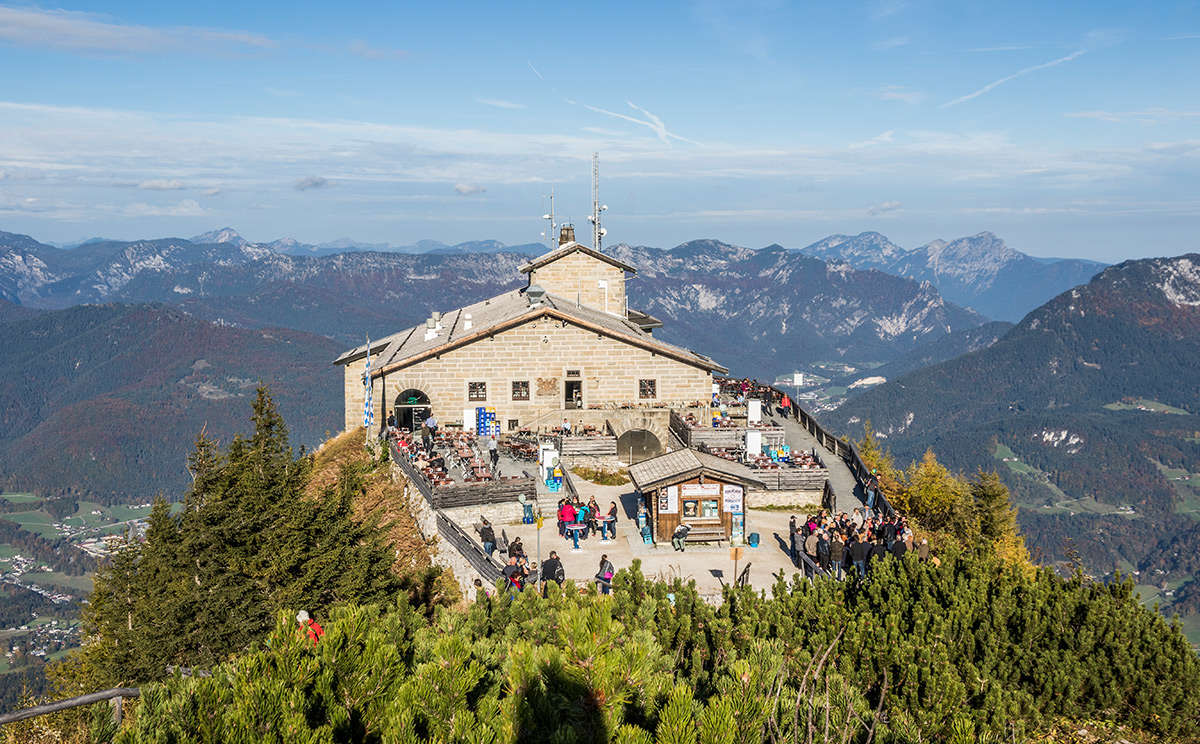This aerial image showcases a central tan brick building with a beige-gray roof, situated on a tree-covered hill or mountain top, amidst a scenic, lush green landscape. The building features a spacious patio or courtyard area, bustling with dozens of people, some sitting at tables and eating, suggesting the presence of an attraction or viewpoint. Adjacent to the main building, there's a smaller wooden structure that resembles a visitor's stand or shop. Surrounding this area are numerous trees, contributing to the verdant setting. 

In the broader view, we see a row of snow-capped mountains in the background, with another distant row that may have a rocky appearance or additional snow. To the left and right of the image, hills are visible. The bottom left corner of the image depicts a small village with some vehicles parked below, while the bottom right also shows additional buildings. The sky above is a bright blue with scattered clouds. Notably, the central building is equipped with radio antennas and satellite dishes, adding to its detailed characterization as a potential viewpoint or attraction site.